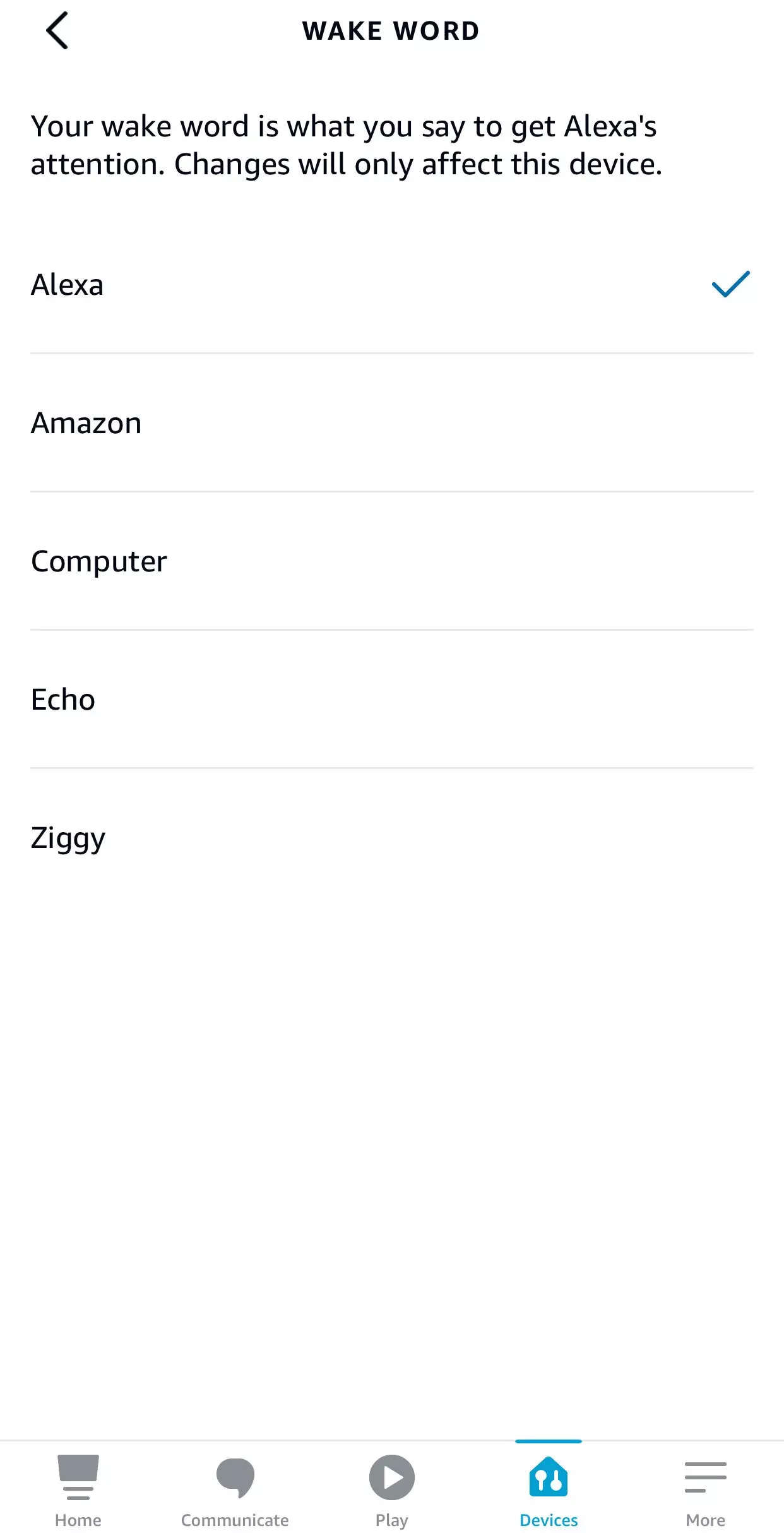This cropped screenshot showcases a partial view of an Alexa settings tab within a mobile app. The top of the phone screen is visible, featuring a bold "Wake Word" header centered at the top. To the left of the header, there is a back arrow icon indicating navigation.

Beneath the "Wake Word" heading, explanatory text reads: "Your wake word is what you say to get Alexa's attention. Changes will only affect this device.” This clarifies the function of the wake word for the user.

Below this description, the screen displays a vertical list of wake word options. The first option, "Alexa," is currently selected, indicated by a checkmark to its left. This selection signifies that the device will respond when the user says "Alexa."

The remaining wake word options are listed as follows:
1. Amazon
2. Computer
3. Echo 
4. Ziggy

The end of the list features an error message: "Boom, boom, boom isn't responding. Please check its network connection and power supply."

At the bottom of the screen, a navigation bar presents four icons: Home, Communications, Play, and Devices. The "Devices" icon is selected and highlighted in blue.